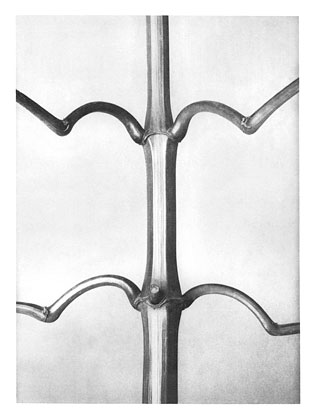The image depicts a vertically oriented, metallic object resembling a bamboo stalk, set against a light gray, almost whitish background. The object features cylindrical sections with alternating thin and thick areas, giving it a segmented appearance. There are two prominent sets of protrusions extending from either side of the central stalk. The top set of protrusions zigzag out from the right and left, forming sharp, angular bends. The lower set of protrusions curves gently to the sides in a smoother, hump-like shape. The metal surface of the object is shiny and reflective, contrasting starkly with the muted, monochromatic background. The overall composition suggests that this is a close-up of a fabricated item that combines organic shapes with industrial materials.